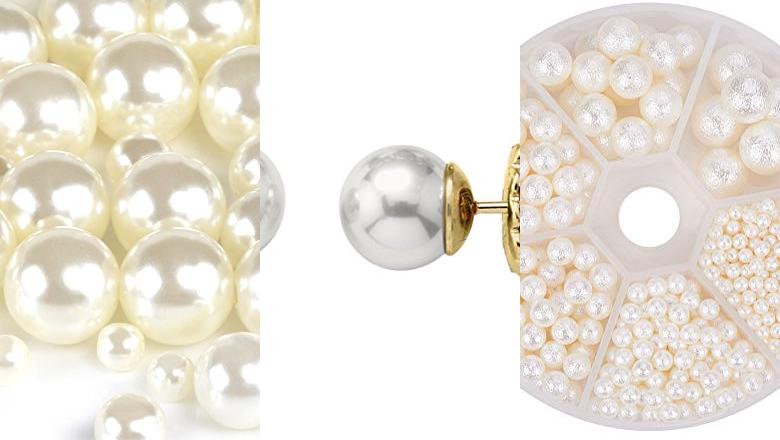The image is divided into three distinct sections showcasing an assortment of pearls. The leftmost section is a close-up of variously sized shiny white pearls scattered on a white surface, with the larger pearls being more prominent among some smaller ones. The center section highlights a practical application of the pearls, featuring a single pearl affixed to a gold earring stud that extends from the right side into the left. The rightmost section depicts a circular storage tray, resembling a Trivial Pursuit game piece, with six triangular compartments each holding different sizes of pearls—from tiny BB-sized ones to larger marble-sized ones. The overall background of the image is white, accentuating the lustrous white of the pearls and the gold of the earring stud.